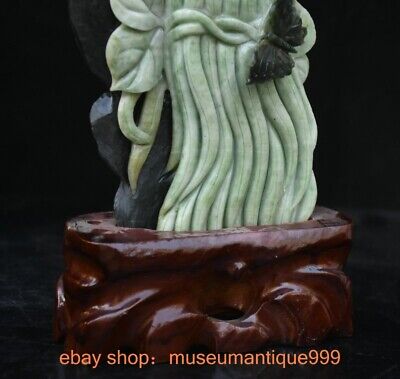This is a detailed photograph of a sculptural artwork. The sculpture features a reddish-brown base with wavy contours that resemble carved wood, supporting an ovular shape with irregular carvings. Extending from this base is a section that emulates a bundle of green plants, meticulously carved and resembling strands of light green marble. At the top right of this green part sits a black butterfly, seemingly crafted from the same material. The sculpture is set against a black background. Beneath the artwork, in pink or orange lettering, are the words "eBay shop: Museum Antique 999."